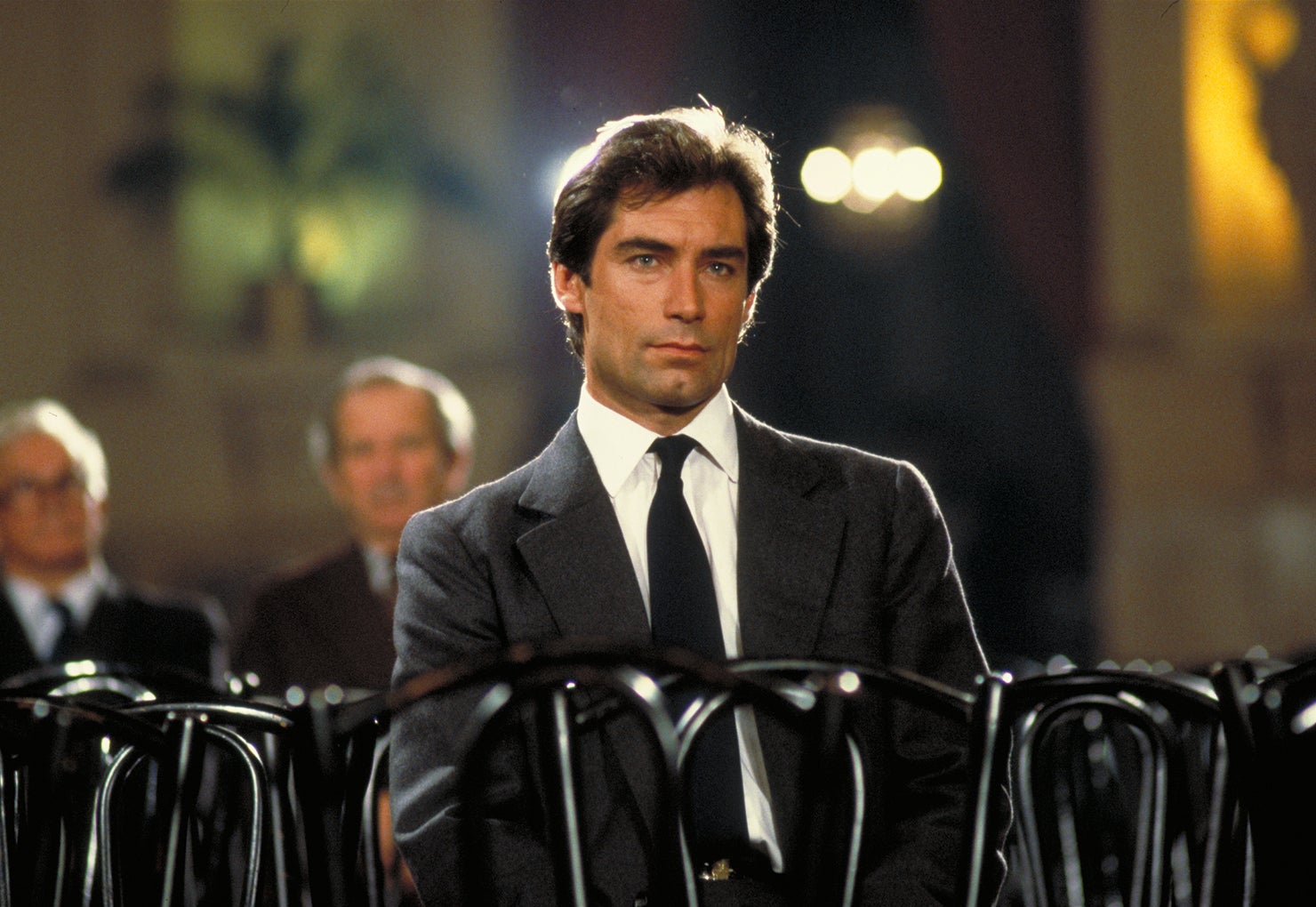In the photograph, a very handsome gentleman with dark brown, well-groomed hair and light-colored blue eyes is sitting on a black metal chair, surrounded by rows of identical chairs. He is impeccably dressed in a dark-colored suit, a white button-down shirt, and a dark tie, exuding a serious and neutral expression with a notable dimple in his chin. His eyebrows are heavy and dark, complementing his straight nose and clean-shaven face.

The image primarily showcases this man in sharp focus, while the background remains blurred. To the left of the man, two older gentlemen, also in business suits, are sitting out of focus. One of these men is bald and wears glasses. Behind the main gentleman, hazy green lights and a goldish-colored light cast a soft, out-of-focus glow, contributing to the subdued ambiance. Part of a plant with green leaves and other abstract elements like a door or walls can also be made out in the blurred background, adding depth to the setting. 

Overall, the scene conveys an atmosphere of quiet anticipation or reflection, with the focused details on the central figure and the blurred, indistinct background enhancing the impression of solitude amidst formality.